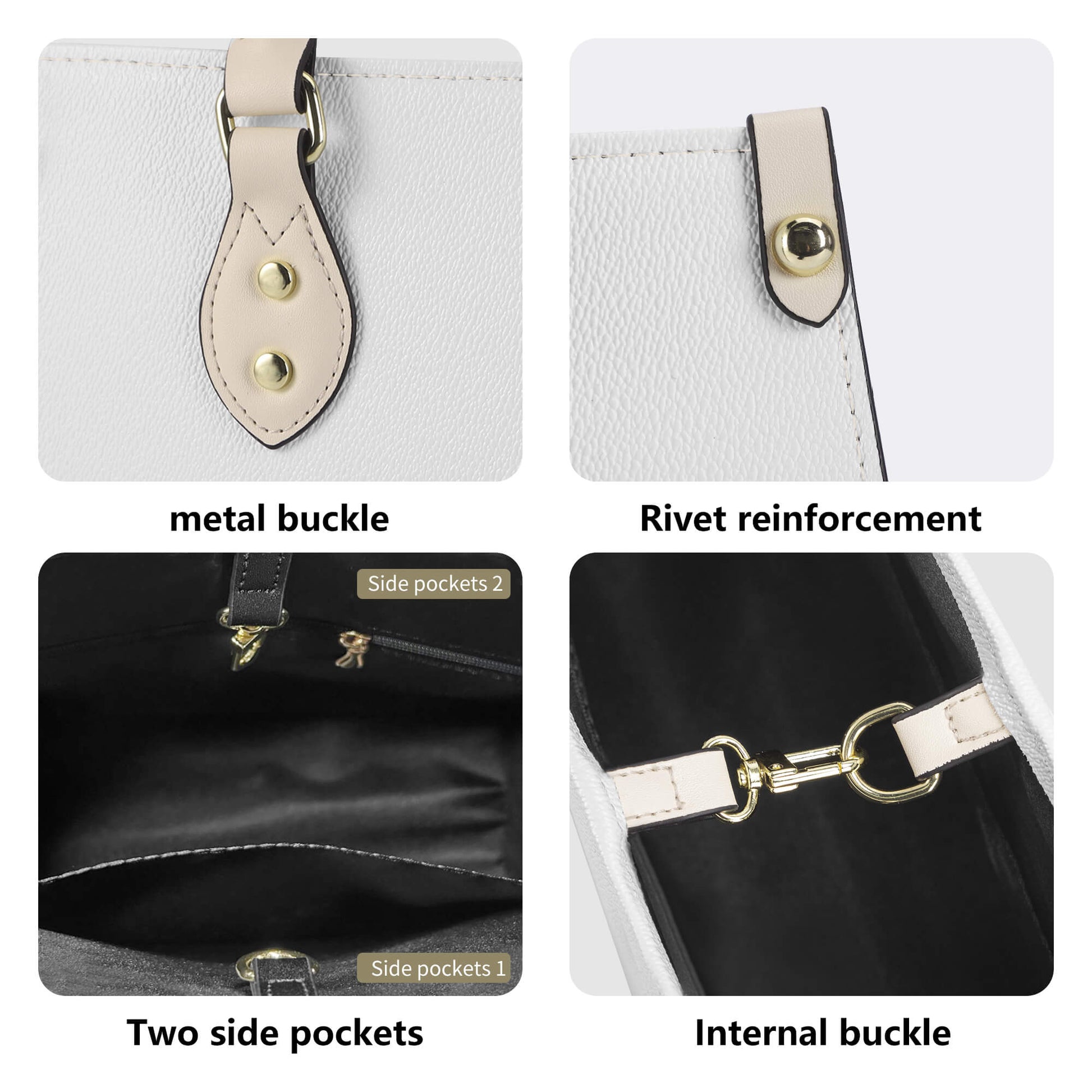The image is a split collage consisting of four distinct photos, each labeled with black text that highlights specific features of various purses. The upper left square showcases a close-up of a white purse featuring an ivory-colored metal buckle with gold accents, labeled as "metal buckle." To its right, the upper right square displays the corner of the same white purse, marked as "rivet reinforcement," emphasizing its durable design. The lower left square presents a detail shot of black fabric accompanied by a zipper, indicating the presence of "two side pockets." Lastly, the bottom right square focuses on another black purse, showing two white latches connected by bronze chain links, labeled as "internal buckle." Each segment of the image meticulously dissects the purse's detailed features, including buckles, pockets, and reinforcements.